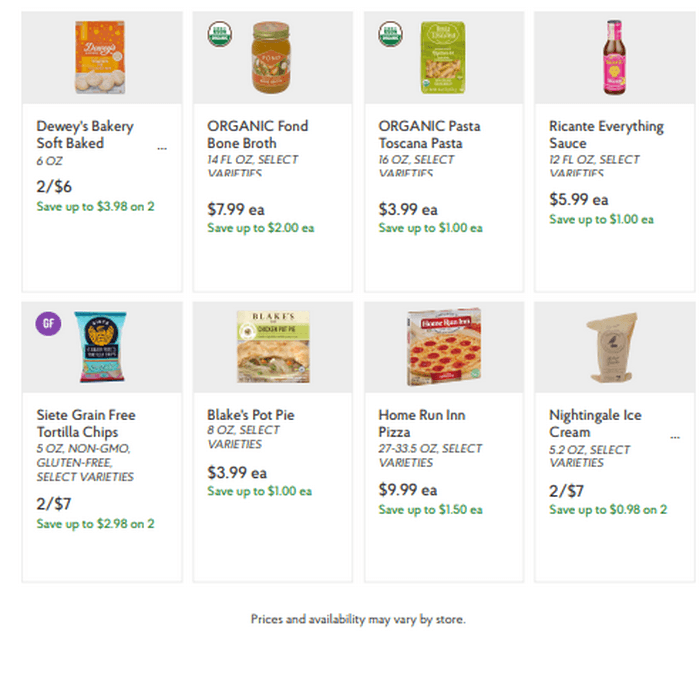**Screenshot from Grocery Web Page:**

The screenshot displays eight light gray colored squares, each containing a distinct food item along with descriptive text. Below is a detailed description of each item from left to right, top to bottom:

1. **Top Left Corner:**
   - **Food Item:** Dewey's Bakery Soft Baked Cookies
   - **Weight:** 6 oz
   - **Price:** $2.06
   - **Savings Offer:** Save up to $3.98 when you buy two

2. **Top Row, Second from Left:**
   - **Food Item:** Organic Fond Bone Broth
   - **Volume:** 14 fl oz
   - **Varieties:** Select varieties
   - **Price:** $7.99 each
   - **Savings Offer:** Save up to $2.00 each

3. **Top Row, Third from Left:**
   - **Food Item:** Organic Pasta Toscana
   - **Weight:** 16 oz
   - **Varieties:** Select varieties
   - **Price:** $3.99 each
   - **Savings Offer:** Save up to $1.00 each

4. **Top Right Corner:**
   - **Food Item:** Ricanti Everything Sauce
   - **Volume:** 12 fl oz
   - **Varieties:** Select varieties
   - **Price:** $5.99 each
   - **Savings Offer:** Save up to $1.00 each

5. **Bottom Left Corner:**
   - **Food Item:** Siete Grain-Free Tortilla Chips
   - **Weight:** 5 oz
   - **Attributes:** Non-GMO, Gluten-Free
   - **Varieties:** Select varieties
   - **Price:** 2 for $7.00

The items are neatly arranged in a grid and each one is accompanied by detailed product information, including weight or volume, pricing, select varieties, and any savings offers available.